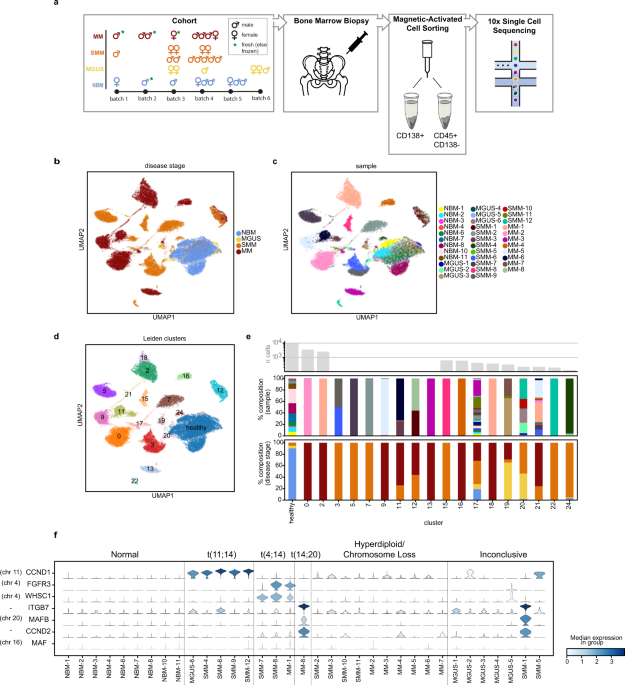The image is a complex assembly of various graphs, charts, and drawings, all organized into labeled sections A through F. The background is white, and the visual hierarchy is structured with A and F occupying the top and bottom portions, respectively. B, C, D, and E are arranged in the middle, with B and C next to each other, as well as D and E.

At the very bottom, section F features a long rectangular graph resembling a table with numbers and words, providing detailed explanations. Above it, section E contains a colorful bar graph with two levels of bars fluctuating up and down, labeled with numbers and various colors.

Section D, positioned above E, showcases a colorful map-like breakdown. Nearby, section C depicts another map-like graph. Right next to it, section B features a square chart with multiple substances labeled according to a color chart, including NBN, NGUS, 5MM, and MM.

The topmost section A contains four rectangular graphs. The leftmost rectangle presents a graph illustrating male and female symbols in blue, brown, and yellow, labeled as "cohort." An arrow points from this graph to the right, leading to a square with a drawing of a bone structure labeled "bone marrow biopsy." Further to the right, another rectangle titled "magnetic activated cell sorting" displays tubes full of liquid. The final arrow points rightward to a rectangle with blue pathway-like lines labeled "10x single cell sequencing."

Scattered throughout the image are additional elements, including a depiction of part of a skeleton with a needle shot, further emphasizing the medical and scientific context of the visualization.